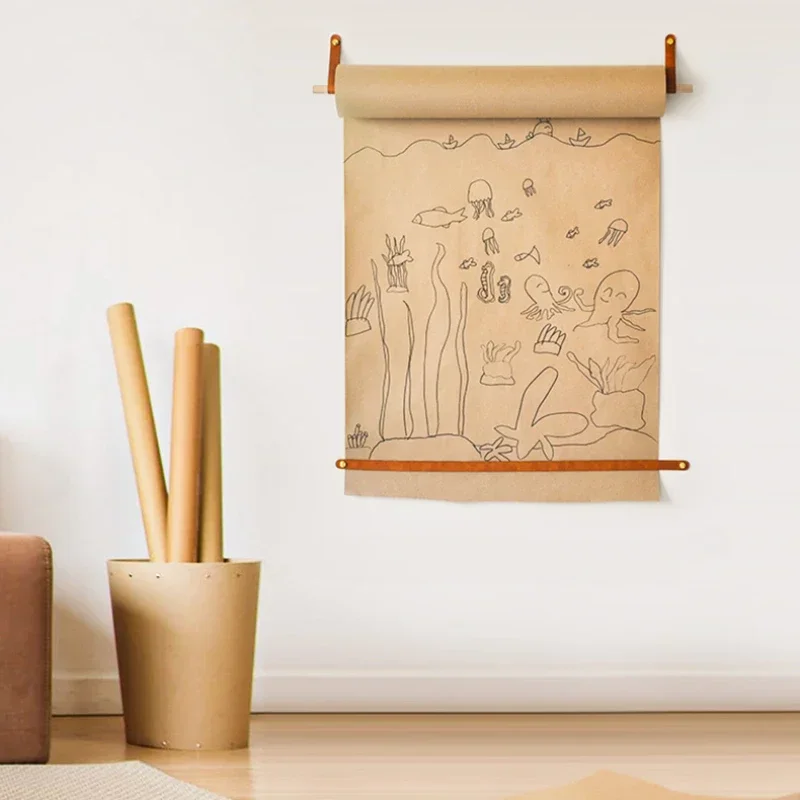This photograph captures a quaint scene of a children's art corner. Dominating the white wall is a large scroll made of beige parchment paper, unrolled and secured at the top with two brown leather straps and hooked on a rod, while a thin wooden strip at the bottom keeps the paper from curling. The scroll features an intricate pencil drawing of an undersea world, including waves with sailboats, and various marine life such as fish, octopuses, seahorses, jellyfish, seaweed, and starfish populating the ocean depths. The setting is grounded by a light brown wooden floor. To the left of the drawing, a brown bucket sits on the floor, filled with three rolls of construction paper, contributing to the creative, artistic atmosphere of the space.